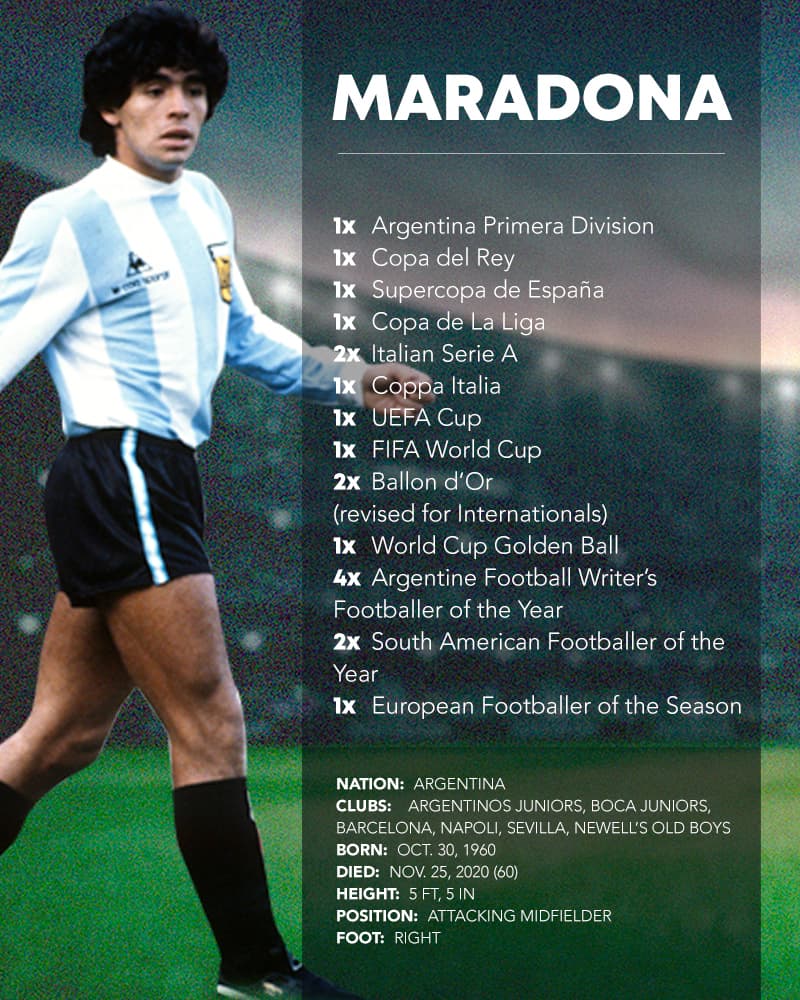This image is a detailed poster of the legendary soccer player, Diego Maradona, providing an in-depth look into his career and achievements. The poster is in portrait orientation and features a youthful Maradona on the left third. He dons his Argentina national team uniform, which comprises a blue and white vertically striped jersey, black shorts with a white stripe down the sides, and high black knee socks. Maradona's dark, full hair reflects the popular style of the 70s and 80s, complete with a loose, slightly pulled-back appearance. He stands on a green field with a mountain in the background, exuding the aura of a rising star in soccer.

The right third of the poster highlights various statistics and accolades associated with Maradona. At the top, "Maradona" is boldly printed in white capital letters. Below, it lists essential details: his nation (Argentina), clubs he played for (Argentinos Juniors, Boca Juniors, Barcelona, Napoli, Sevilla, Newell's Old Boys), his birth date (October 30th, 1960), and his death date (November 25th, 2020). It also specifies his height (5'5"), his position (attacking midfielder), and his dominant foot (right). Additionally, the poster enumerates his significant accomplishments, including his World Cup and UEFA Cup victories, accentuating the legendary status that immortalized him in the world of soccer.